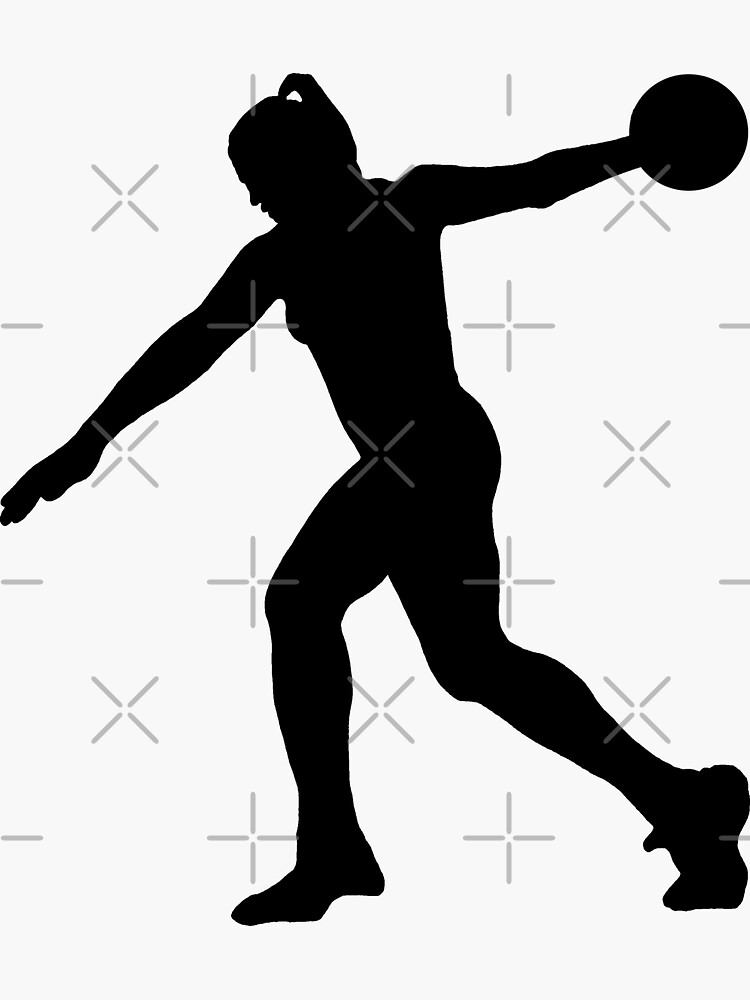The image displays a highly detailed black silhouette of a muscular female athlete against a predominantly white background. The figure, featuring a ponytail and identifiable breast outline, takes up most of the frame. She stands poised with her right arm extended forward, palm facing down, and her left arm raised behind her, holding a large ball or disc. Her athletic build is accentuated, and she appears to be wearing gym shoes with a notable long tongue on one of them.

The backdrop is distinguished by an intricate grid pattern formed by evenly spaced gray Xs and dotted lines, dividing the background into nine distinct sections. These Xs and crosses are slightly transparent, overlaid meticulously on the white canvas, creating an impression of precision and symmetry. The artistic rendering of the image resembles a rotoscoped or traced photograph, highlighting the athlete's form and stance in stark contrast against the grid-patterned white background.